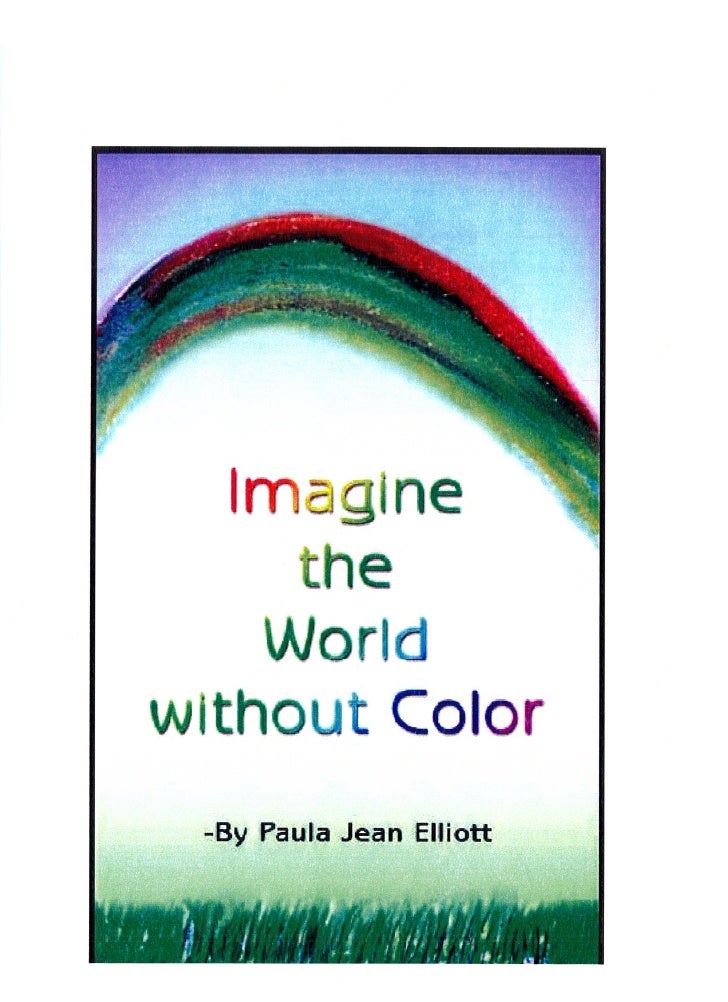The image appears to be a book cover or possibly a graphic visible on a computer screen, designed in a painterly illustration style. Dominating the upper portion, a gradient sky transitions from deep purple at the top to lighter blue near an arching rainbow. This rainbow features unusual hues, including red, black, dark green, lighter green, brown, and lime green.

Below the rainbow, text with a multicolored "Imagine" stands out, each letter colored distinctly in red, yellow, green, and lime green. Following this, the word "Dirt" appears in green, and beneath that, "The World" is portrayed with "WOR" in green and "LD" in blue. The phrase "without color" follows, rendered in grayscale with no color.

At the bottom, the artwork credits Paula Jean Elliott, and hand-painted green grasses rise toward the rainbow, completing the composition with a sense of natural growth and vibrancy. The layout is rectangular and in portrait orientation.

The core message conveyed is "Imagine the World Without Color," encapsulated by vivid and contrasting elements throughout the design.